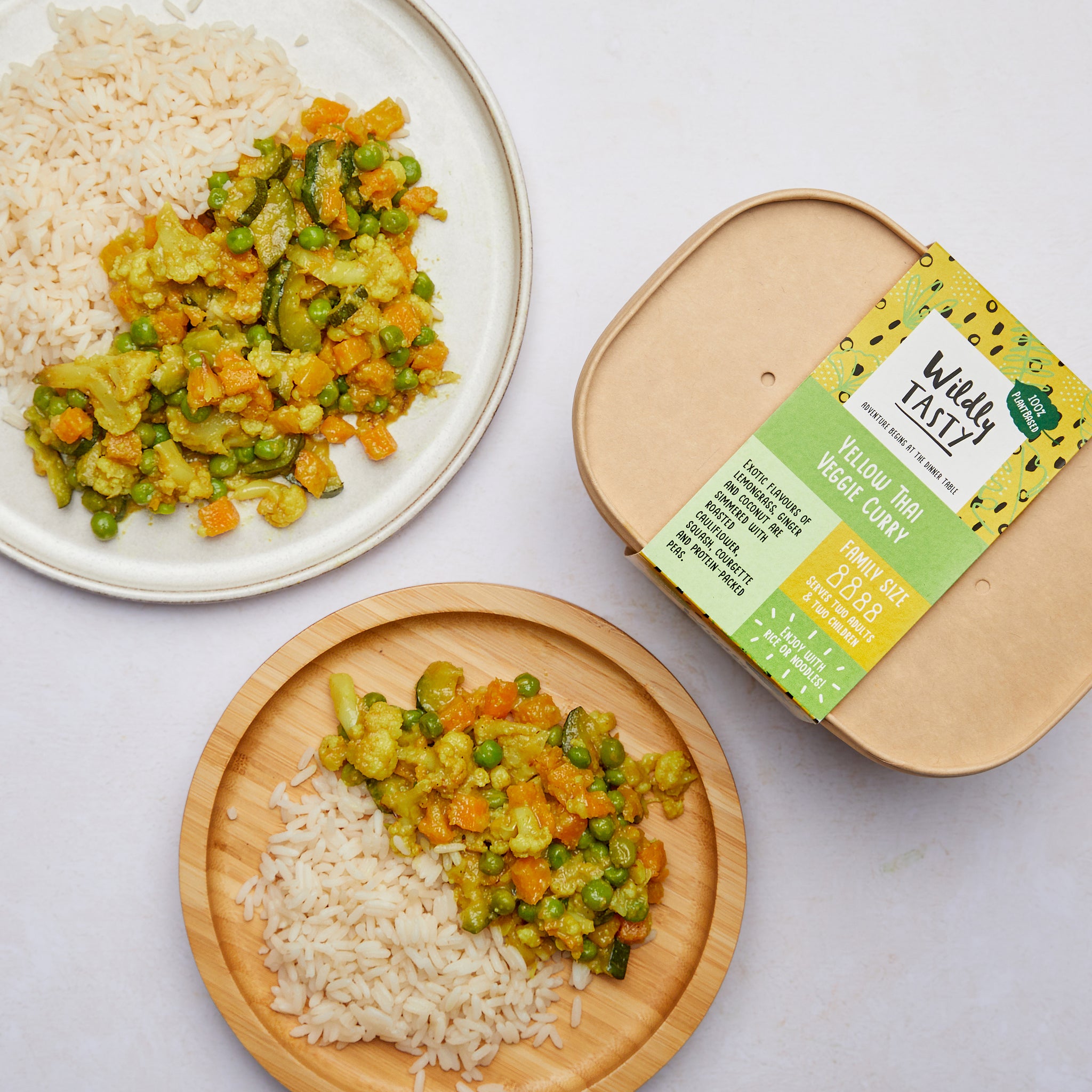The image features three items: two plates and a wooden package. The wooden package resembles a bowl with a Tupperware-like appearance and has a paper label wrapped around its center. The label reads "wildly tasty yellow Thai veggie curry." The two round plates, one white and the other wooden, both display servings of yellow Thai veggie curry accompanied by a portion of white rice.